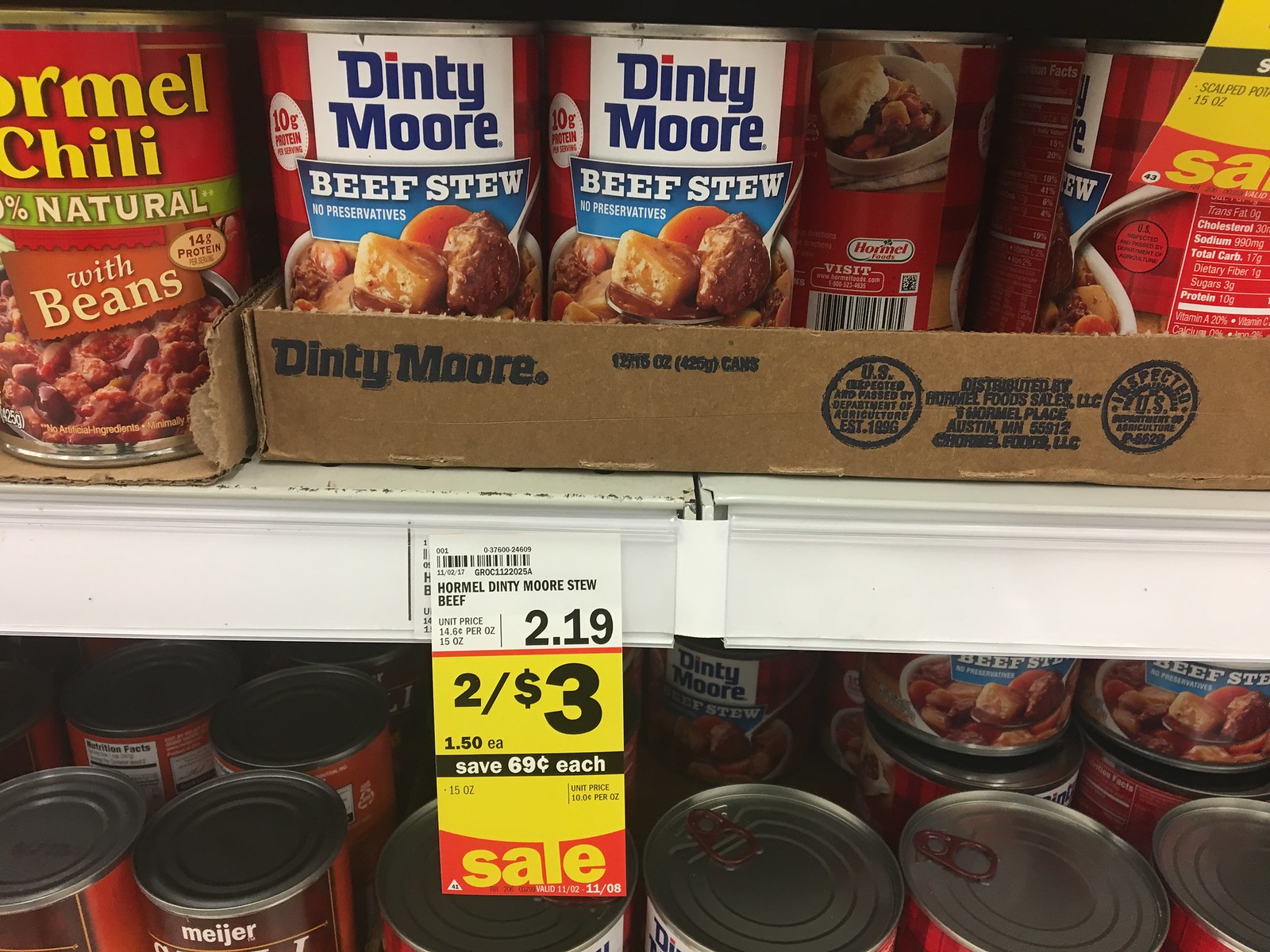The image is a close-up, landscape-oriented photograph of a couple of shelves in what appears to be a North American supermarket or grocery store. The top shelf prominently displays canned goods, specifically Hormel chili and Dinty Moore beef stew. The Hormel chili cans feature yellow text that reads "With Beans" and an image of a bowl of chili. Next to them, the Dinty Moore beef stew cans are labeled with blue text on a white background stating "No Preservatives" and showcasing a bowl of beef stew with a spoon.

On the top shelf, the price tags are clearly visible. A label within a plastic edging shows a promotion: two cans for three dollars, with an additional note indicating a single can costs $1.50 each. Below the price, a red tag with yellow writing announces a sale, stating "SAVE 69¢ each." Some cans rest in a cardboard box lid labeled "Dinty Moore."

The bottom shelf, partially visible, holds more canned beef products, including a brand labeled "MEIJER." Unlike the top shelf, branding and additional details on the cans on the bottom shelf are not fully visible due to cropping. The pricing and promotional information further confirm the North American setting with the usage of the dollar sign and familiar grocery store sale signage.